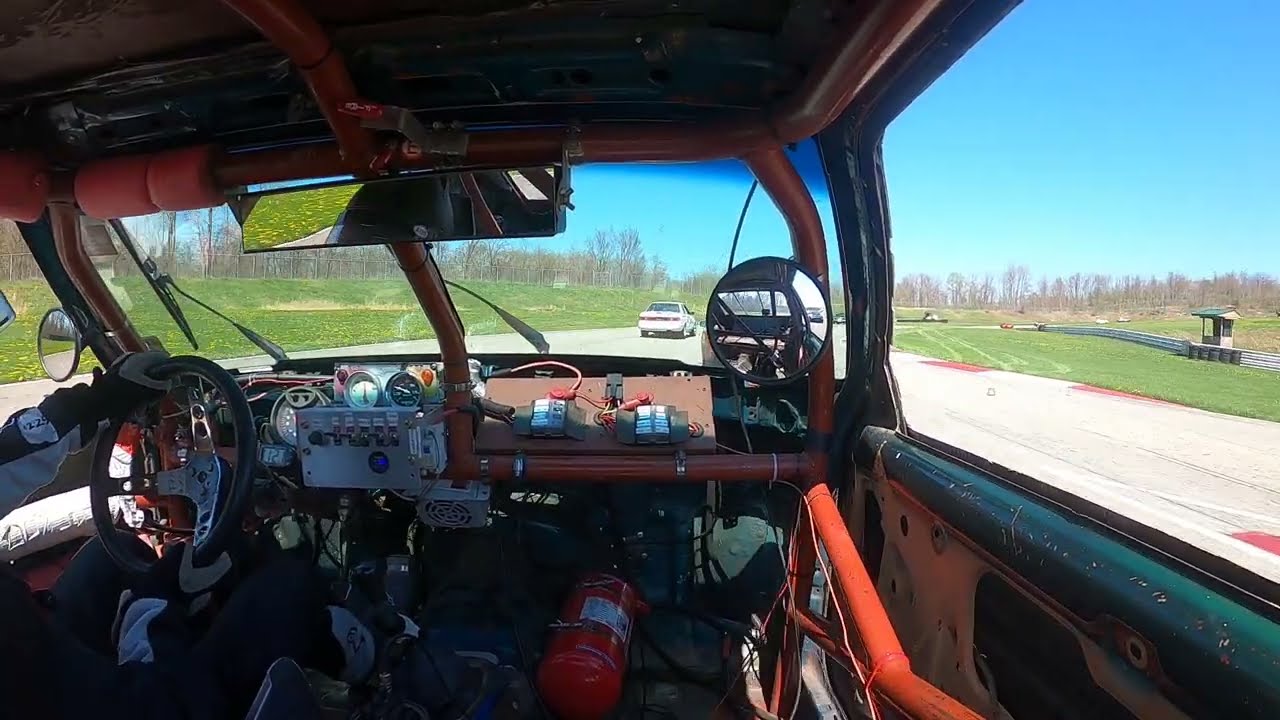The image captures the detailed interior of a race car in the midst of a drive on a closed track, likely during winter given the leafless trees visible outside. The setting is bathed in daylight with a clear, turquoise sky overhead. Inside the car, a driver, dressed in racing attire and gloves, grips a black steering wheel. The race car's unconventional design features wide or possibly open windows, and the framework is dominated by a sturdy orange roll cage, designed to protect the driver in case of a rollover.

Within the driver's field of view, multiple gadgets, including a round rear-view mirror on the right and a larger rectangular rear-view mirror on the top center, provide essential visibility. A red fire extinguisher is positioned where a passenger's legs would typically be, underscoring the car's safety measures. Additionally, numerous cables and racing tools are scattered inside the vehicle, highlighting its specialized nature.

The scene outside the car extends to a racetrack with white pavement, curving to the right ahead. Surrounding the track are green grassy areas, and ahead of the driver, a white race car can be seen, indicating a competitive race scenario. With the intricate descriptions of objects, colors, and setting, the image creates a vivid portrayal of the race car environment and the dynamic racing context.